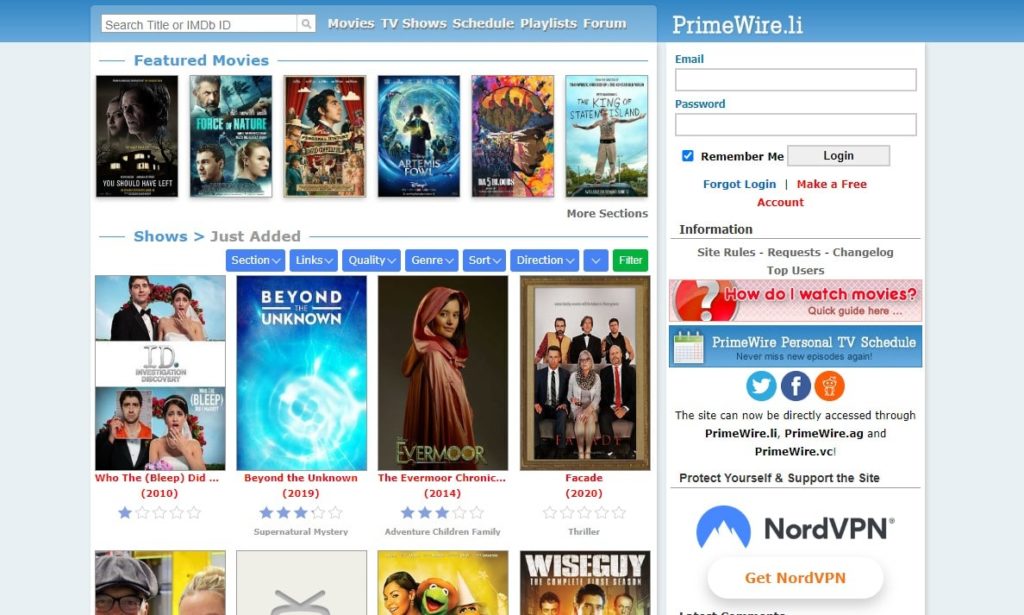This screenshot captures the homepage of the website Primewire.li, which offers a variety of movies and TV shows. 

On the left side of the page, users can see several input fields for login purposes, including text boxes for email and password, along with a "Remember Me" option and an elongated login button to the right of these fields. Below the login section, there is an informational area featuring various tabs such as "Sites," "Rules," "Requests," "Change Logs," and "Top Users." Situated beneath these tabs is a square labeled "Quick Guide," followed by a blue rectangle promoting the "Prime Wire Personal TV Schedule," and three buttons for sharing content on social media platforms: Twitter, Facebook, and Reddit. Further down, there are links to access the site through three different domains and an advertisement for NordVPN.

On the right side of the page, the layout displays numerous movie and TV show posters. The top section is dedicated to movie posters, while TV show posters are organized in the bottom section.